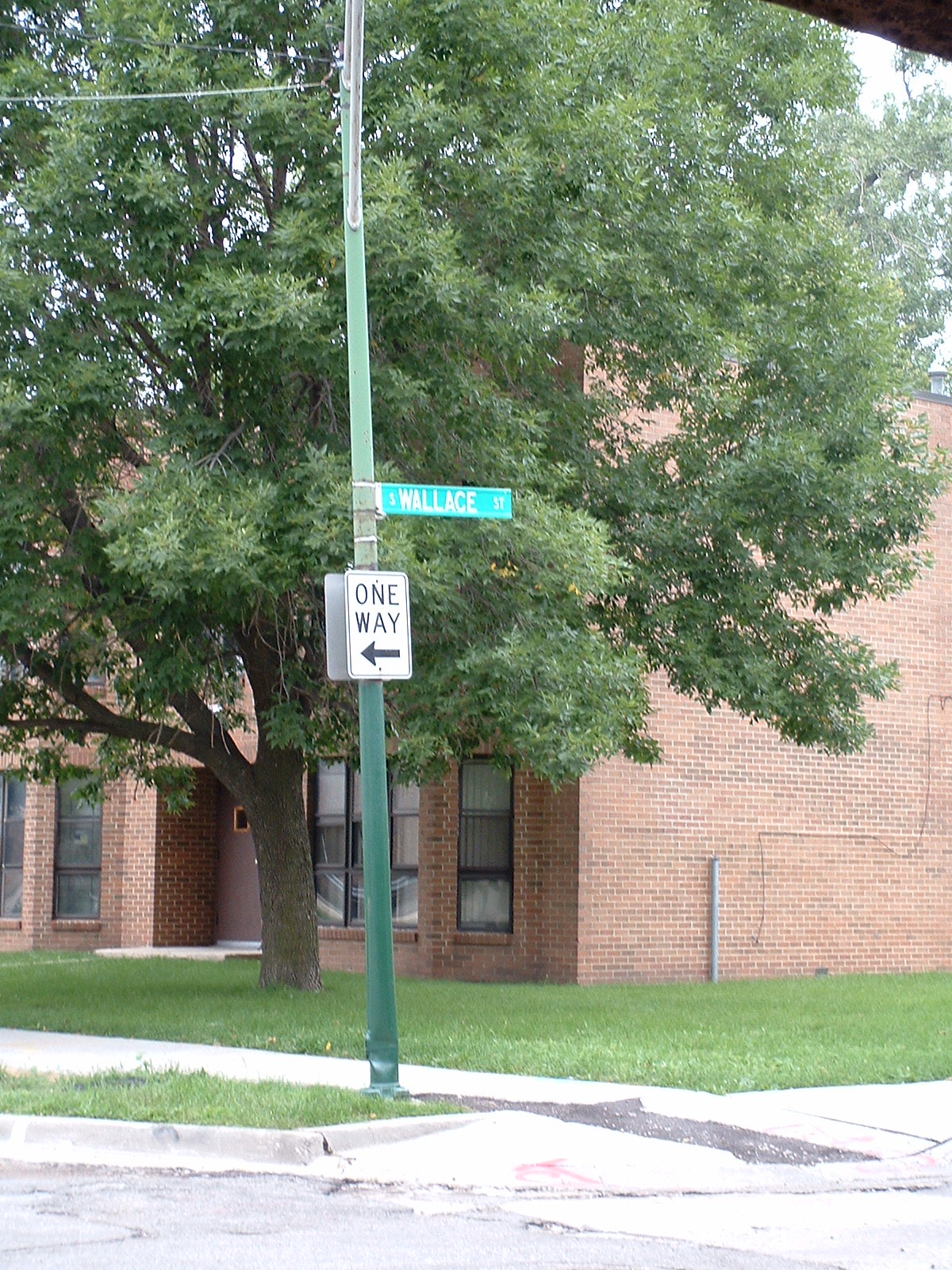This is a detailed color photograph of a street corner, capturing a vivid urban scene. Dominating the foreground is a green signpost bearing two signs. Mounted midway on the pole, a white one-way sign with a black arrow points to the left. Above it, a green street sign with white lettering reads "Wallace St" with "Wallace" in a larger font. The signpost itself transitions from green at the base to nearly white as it ascends. To the left of the sidewalk surrounding the signpost is a lush green lawn with a fully grown, healthy tree, characterized by a thick trunk and numerous branches laden with leaves.

Behind the tree, a red brick apartment building stands prominently. This residential building features a number of multi-pane windows with black surrounds, and a dark brown door that is recessed from the facade, accessed by a single step leading to a small patio area. The sidewalk, light gray in color, stretches along the base of the image, bordered by more grass on either side. To the far left, a portion of the road is visible, while to the right, the sidewalk continues, merging with another. The sky, a light blue, is mostly obscured by the abundant foliage of the tree, providing a tranquil canopy over the scene.